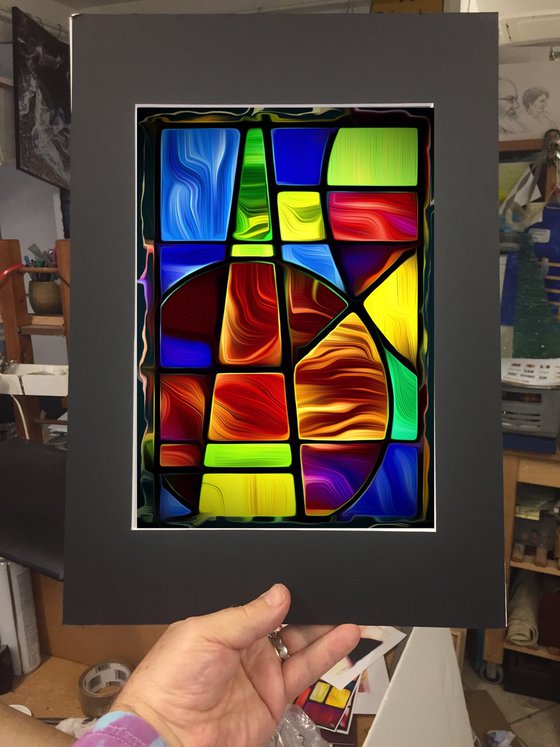In the foreground of the image, a man's left hand, adorned with a silver wedding ring on his marriage finger, holds a vertically aligned rectangular picture frame with a charcoal-colored border. Only a hint of his sleeve is visible at the wrist. The frame showcases an art piece that resembles stained glass, composed of various geometric shapes including trapezoids, triangles, squares, and circles. These shapes are filled with mild but diverse colors like greens, blues, yellows, ochres, browns, and reds. The colors do not harmonize perfectly and some panels feature vertical or horizontal swirls, while others have solid lines. In the background, possibly inside a house, workshop, or art studio, shelves filled with indistinct items and clutter can be seen. There are also white walls adorned with pictures or posters, contributing to the ambiance of a busy creative space.